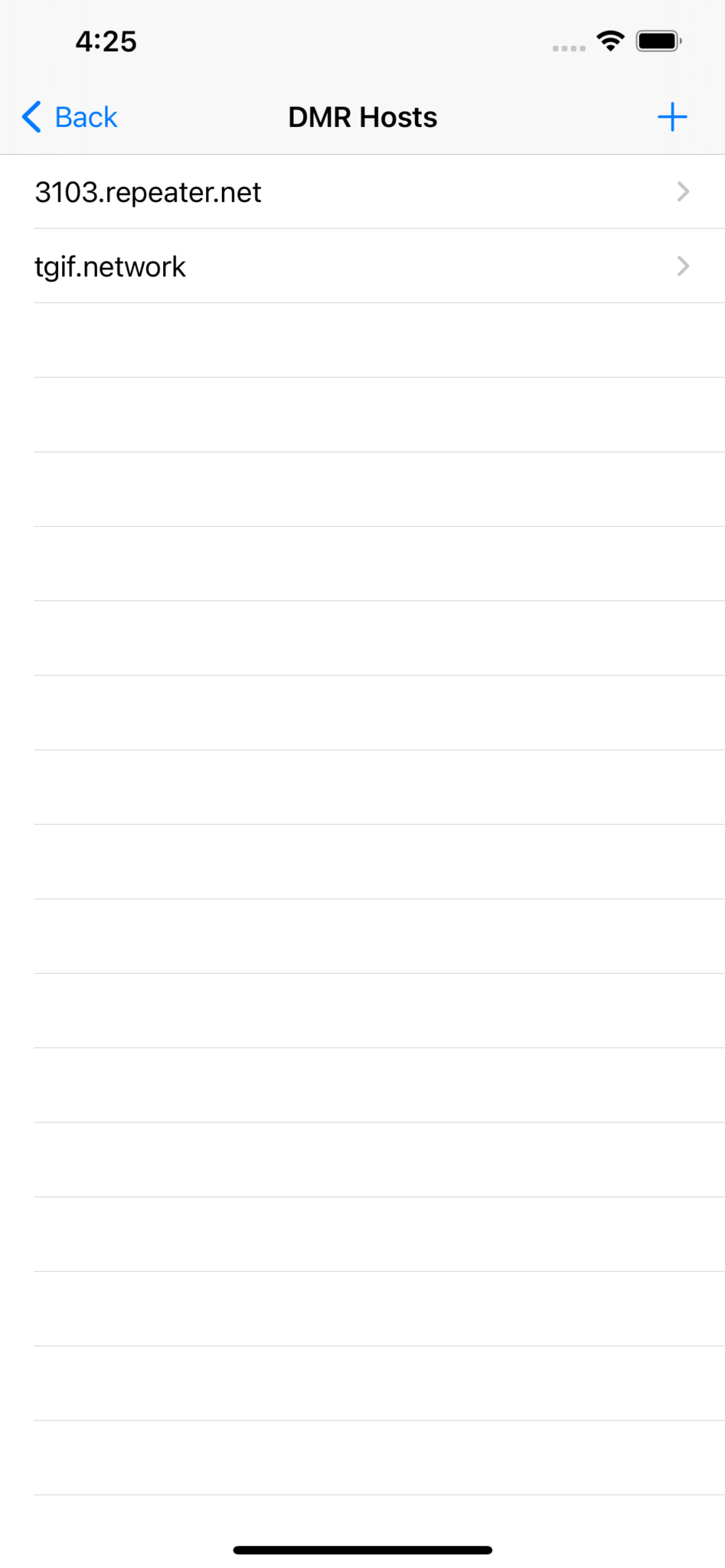The screenshot displays a digital interface with various elements. At the top of the screenshot, the number "425" is prominently visible. Next to this number, there's a "DMR Host" label and a back arrow indicating a navigational option, both colored in blue. Alongside these elements is a blue plus sign, suggesting the ability to add something new.

Below this section, the interface is designed to resemble a notepad, featuring several lines for information input. On the first line, there is the text "3103.repeater.net" followed by a rightward-pointing arrow in light gray. Directly beneath this, on the second line, the text "TGIF.network" is displayed, also accompanied by a light gray rightward-pointing arrow. Both sets of text are rendered in black, ensuring clear readability.

Towards the bottom of the screenshot, a notable black horizontal line runs across the middle section, providing visual separation within the interface.